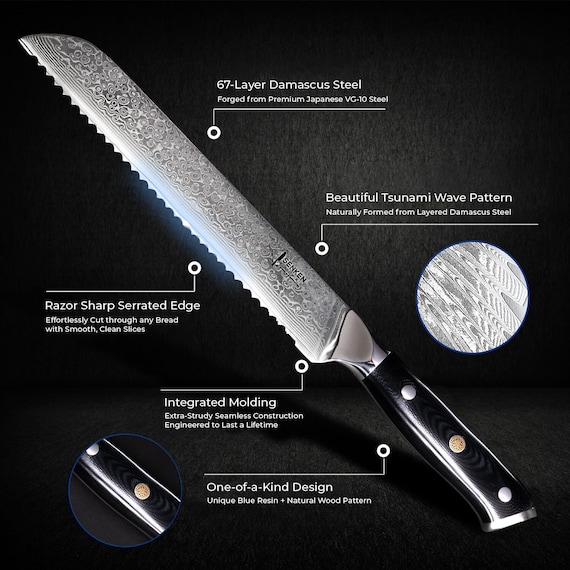The image is a detailed advertisement of a high-quality serrated bread knife set against a deep, black background. The knife is placed diagonally with the black handle in the bottom right corner and the blade extending toward the top left. The handle is embellished with three silver pins, the middle one being more ornate than the others, and features an integrated molding design for extra sturdiness and seamless construction. The base of the handle is silver, and from there, the blade begins with a bit of exposed silver tang. 

The blade itself is made from premium 67-layer Damascus steel, known for its razor-sharp, serrated edge, which effortlessly slices through bread. It showcases a beautiful tsunami wave pattern that results naturally from the layering process. The advertisement includes white-lettered annotations positioned with arrows pointing to various features of the knife. 

To the right of the knife, at the top of the handle, a small circle contains a zoomed-in view of the blade, highlighting the intricate wave pattern. Additionally, in the bottom left corner, there is another circle with a blue border that provides a close-up view of the handle's unique blue resin natural wood pattern. Arrows beneath the knife point to further descriptive text, elaborating on its craftsmanship and distinctive features.